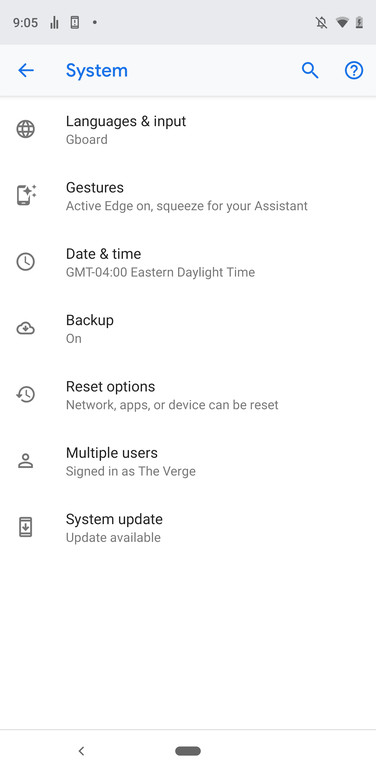The image is a screenshot taken from a cell phone displaying the system settings menu. At the very top, there is a light gray status bar showing the time as "9:05" along with signal strength icons, Wi-Fi connectivity, and remaining battery life. On the right side of this bar, there is a bell icon with a diagonal line through it indicating that notifications are silenced.

Below the status bar, a slightly lighter gray navigation bar is present. It contains several elements: on the left, a left-facing arrow icon, next to the word "System" in blue text with a capital "S". To the right of the text are a magnifying glass symbol, which represents the search function, and a circular icon with a question mark inside, likely indicating help or support options.

The main content of the screenshot displays a list of system settings options, each prefaced by a small icon:

1. **Languages & input**: Displays "Gboard" underneath.
2. **Gestures**: Summarized by "Active Edge on, Squeeze for your Assistant."
3. **Date & time**: Shows "GMT-04:00, Eastern Daylight Time."
4. **Backup**: Indicates that backup is "On."
5. **Reset options**: Describes options to "Network, apps, or device can be reset."
6. **Multiple users**: States "Sign in as The Verge."
7. **System update**: Notes that an "Update available" is present. 

Each option is accompanied by a succinct description of its current status or specific configurable settings.